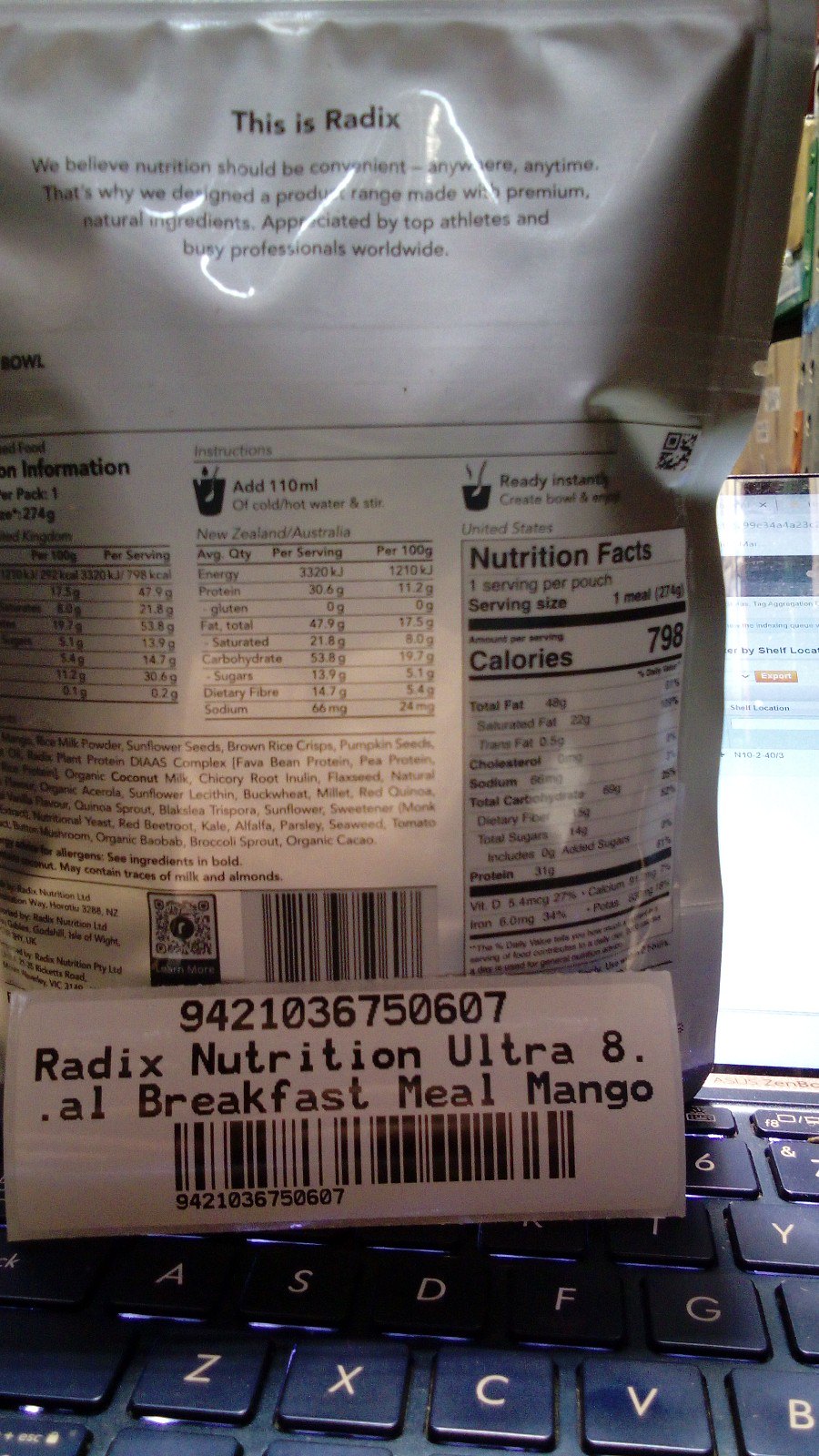The photograph captures a close-up view of the back of a white, shiny plastic package of Radix Nutrition Ultra 8 Breakfast Meal Mango, positioned on a black laptop keyboard with white letters. The package features black print text and a white sticker displaying the serial number 9421036750607, along with a barcode. The sticker includes the product name and type, while the black print above reads, "We believe nutrition should be convenient anywhere, anytime. That's why we designed a product range made with premium natural ingredients appreciated by top athletes and busy professionals worldwide." Below this text, nutritional information is visible, highlighting 798 calories and a lengthy list of ingredients. The laptop keyboard extends vertically, occupying the lower portion of the image, and hints of a blue and white computer monitor screen can be seen in the upper right background.